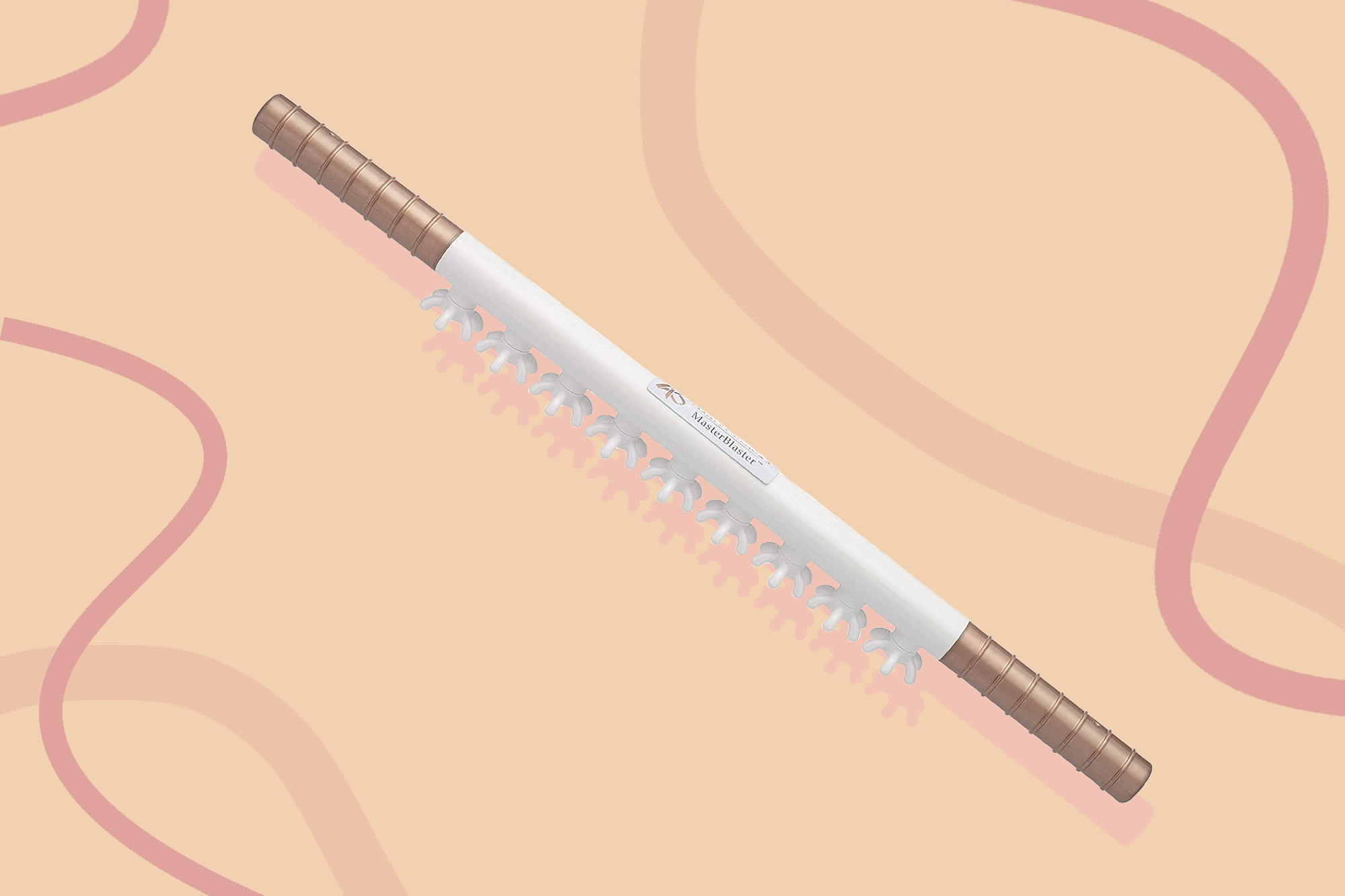The image displays a product prominently positioned diagonally across a beige-pink background with light shadows and reflective highlights. The product, a slender white cylindrical stick with gold-brown threaded ends, features the label "Master Blaster" in the middle. Surrounding the stick are squiggly lines in varying shades of pink and mauve. At the bottom of the stick, there are nine small, leg-like appendages resembling octopus feet. The background's peach and pink hues, along with the delicate lines, add to the distinctive presentation. The product appears to be tilted with its back end pointing slightly toward the top left corner and the front end toward the bottom right.